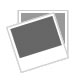In this indoor image, there is a medium brown wooden table with visible wood grains set against a plain white wall. On the table, three distinct items are arranged. Firstly, there's a can of Campbell's condensed tomato soup, featuring the iconic design with a red upper half, the white Campbell's logo, and a white lower half bearing the words "tomato soup" along with a central gold circle. Adjacent to the can is a shiny, golden-colored cylindrical object with varying sections, similar to a telescope end, and a side dial with illegible text. This metallic decor piece stands on a round gray base. Lastly, to the right of the cylindrical item, a bronze lion figurine is mounted on a small black platform. The objects cast faint shadows on the white backdrop, enhancing the image’s realistic indoor setting.